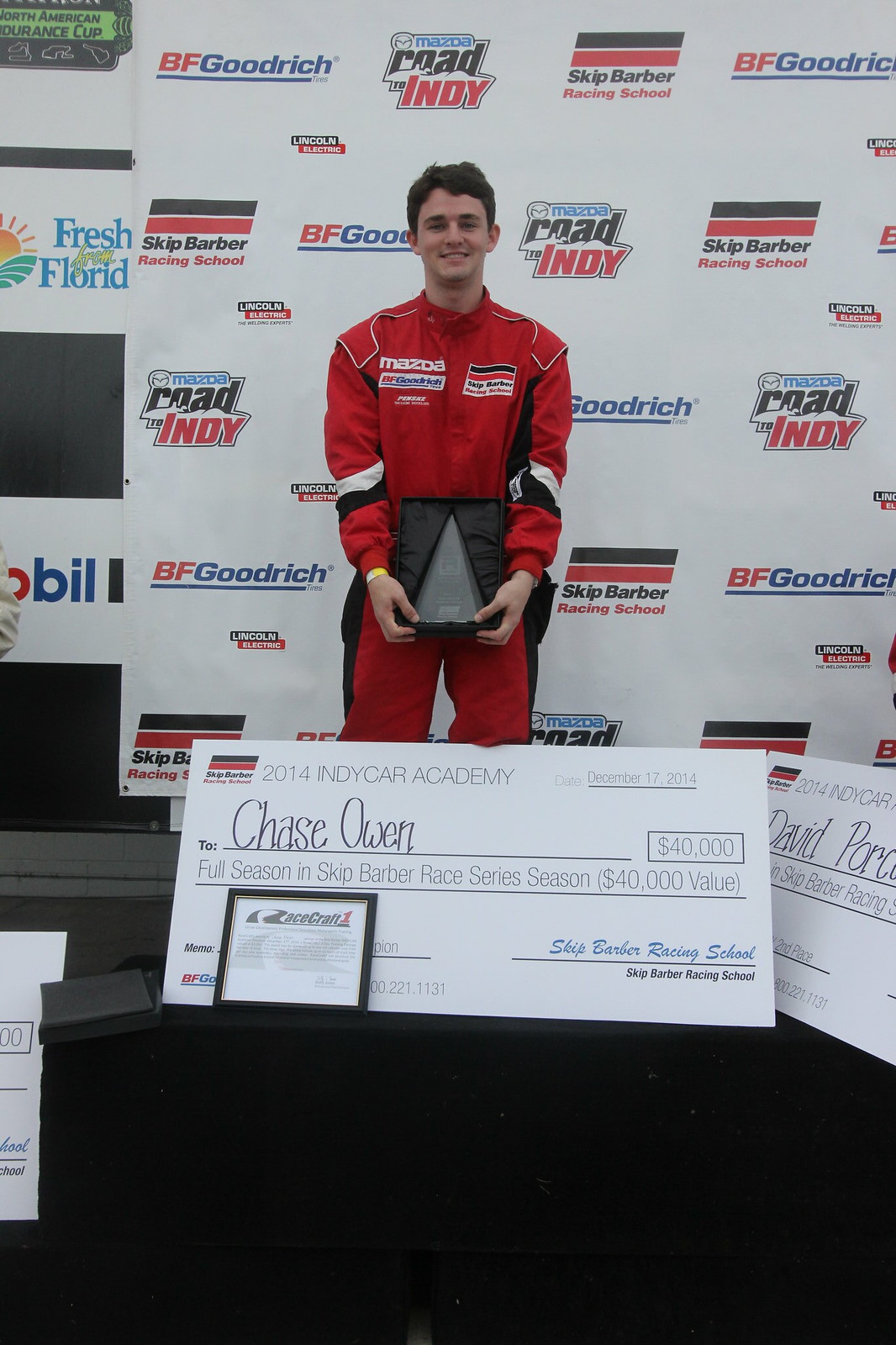The image is a horizontally rectangular, full-color photograph likely taken indoors judging by the lighting. It features Chase Owen, a white male, standing proudly. He is dressed in a red racing suit adorned with a Mazda sponsor logo. In front of him, he holds an oversized check for $40,000 awarded by the IndyCar Academy as well as a triangular-shaped trophy, and he is smiling warmly at the camera. The backdrop consists of a wall covered in a sheet displaying various sponsor names in white, red, blue, and black colors, including BF Goodrich, Mobil, Fresh Florida, Skip Barber, and Mazda. The scene showcases Chase Owen's significant achievement, framed by the celebratory sponsor-laden backdrop.